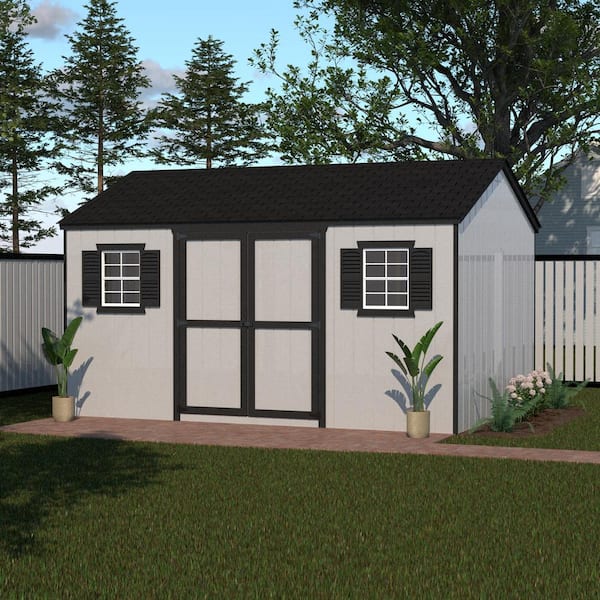This vibrant color illustration depicts a quaint backyard scene featuring a charming shed. In the foreground, a lush green lawn extends to a neat little brick walkway that leads up to the shed set further back. The shed is the focal point of the illustration, with a light gray exterior and a sturdy black roof. It has two central doors with black frames, complemented by small, symmetrical windows on either side. Each window is adorned with white and black frames, highlighting the quaint black decorative shutters.

Nestled at the corner of the shed are two verdant green plants housed in simple planters, adding a touch of nature to the scene. To the right of the shed, colorful flowers flourish in a small brown patch, bringing a splash of color and vibrancy to the composition.

Surrounding the shed is a tall, slatted light gray fence topped with a black trim, providing a sense of privacy and enclosure. Beyond the fence, a towering tree stretches towards the sky, which is painted with soft, fluffy clouds against a serene blue backdrop. The overall scene exudes a peaceful and serene backyard ambiance.